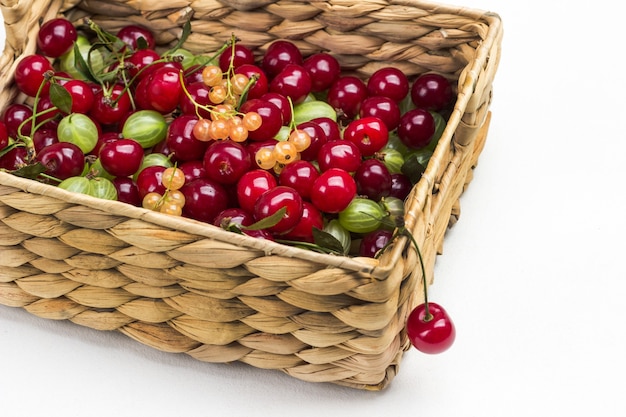The photo features a meticulously arranged basket of various fruits, predominantly vibrant red cherries with shiny green stalks. Approximately two-thirds of the basket's contents are these cherries, which are plump and glossy. The basket itself is a light tan, square-shaped wicker piece, skillfully woven in a cross thatch design, giving it an intricate texture. Nestled among the cherries are about ten gooseberries, characterized by their grape-like shape and light green color, adorned with veiny lines. Additionally, there are smaller, orangey-red berries, possibly currants, adding a splash of variety. A charming detail is a single cherry dangling over the edge, seemingly attempting to escape. The entire arrangement is set against a pristine white background, possibly a table or countertop, enhancing the natural colors of the fruits.